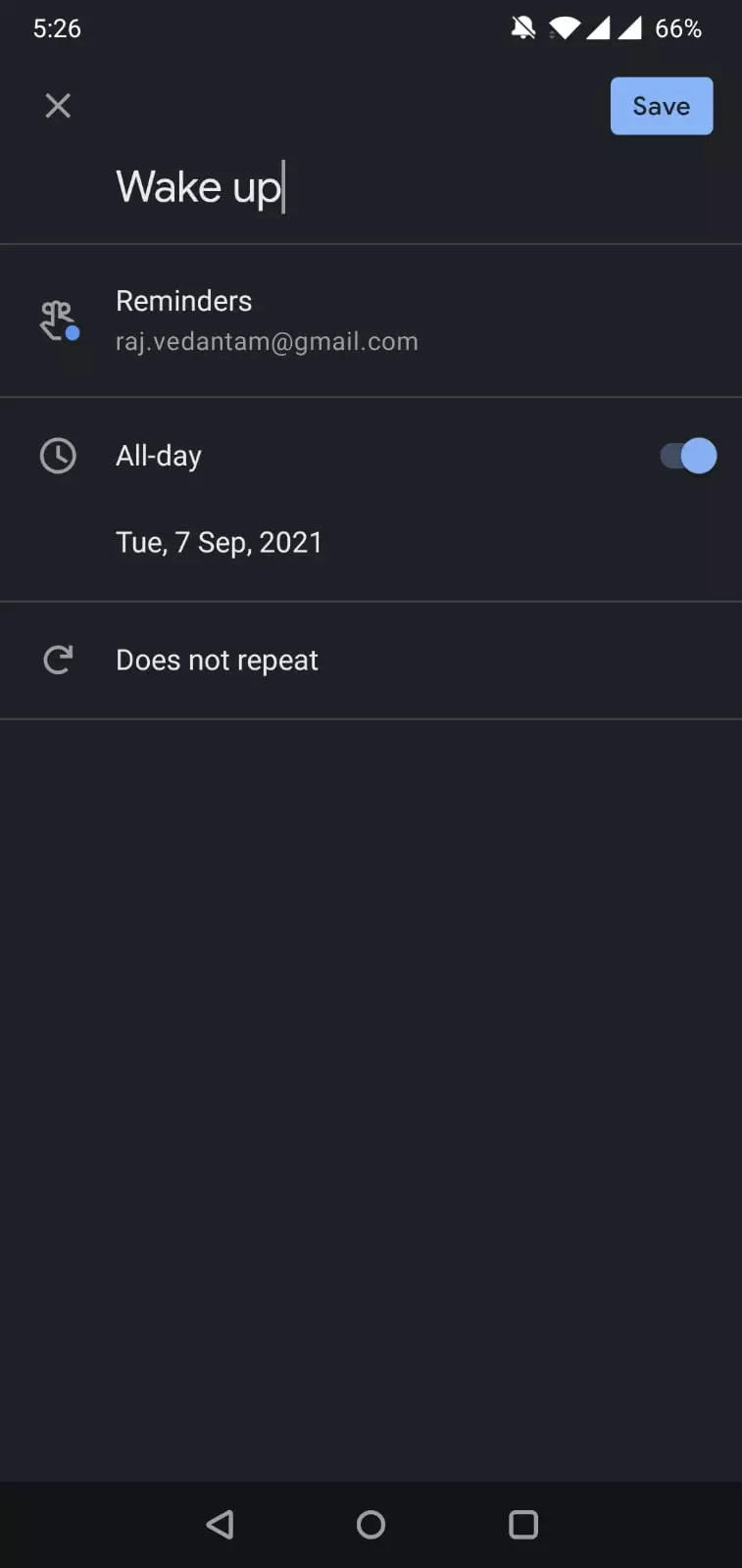### Detailed Caption

This image is a screenshot of a settings page on a smartphone. In the top left corner, the device's time is displayed as 5:26, and in the top right corner, the battery level is shown at 66%. There is also a blue "Save" button located at the top right.

The main header of the settings page reads "Wake Up," with a small cursor line visible after the letter "E," indicating the text might be editable. Below this header, the page is titled "Reminders." The reminder is associated with the email address raj.vedentum@gmail.com.

The settings include an "All Day" option, which is currently toggled on, indicated by a blue switch. Below this, the date is specified as Tuesday, September 7th, 2021, and it is noted that the reminder "Does Not Repeat."

This setup suggests that a reminder is configured for the specified date without a recurring schedule. Although the reminder appears to be set for the entire day, no specific time is provided, implying it could notify the user at the start of the day—midnight—or possibly remain as a persistent notification. The label "Wake Up" hints at a wake-up call; however, it is identified as a reminder rather than an alarm.